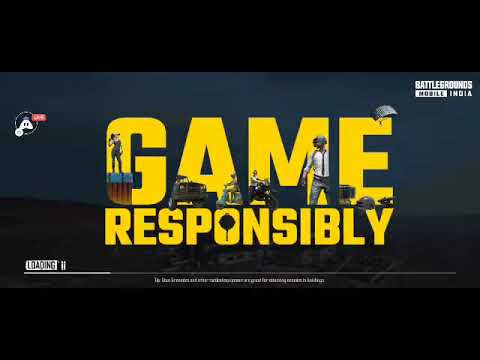The image appears to be a landscape-oriented loading screen for the mobile video game "Battlegrounds Mobile India." Dominating the center are large, bold yellow letters spelling out "Game Responsibly," with various characters and vehicles like an all-terrain vehicle, a scooter, a motorcycle, and a parachuter integrated into the lettering. A progress bar labeled "Loading" is positioned below the text, about a quarter of the way completed. The backdrop is a dark gray-blue landscape, and a horizontal black bar runs across the top and bottom edges of the image. In the top right corner, there is white text that reads "Battlegrounds Mobile India." The image also features an array of subtle colors, including black, green, blue, brown, gray, white, and red, while the bottom of the screen is adorned with some small, unreadable print and a white line.